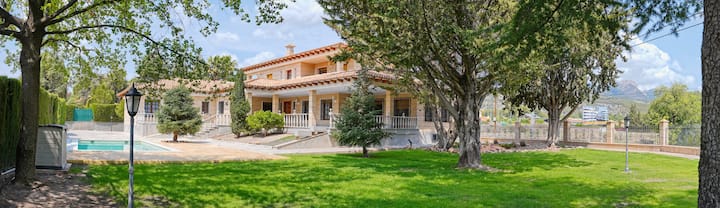This image showcases a spacious, two-story, Spanish-style house with a beige stucco exterior and a brown tile roof. The property features a large, well-manicured lawn with bright green grass and several trees, including a prominent large tree, possibly an oak, and a few smaller ones near the edges. Surrounding the yard is a tall fence with a stone base and metal detailing, complemented by shrubbery that serves as a natural buffer between neighboring properties.

To the left side of the image, a long driveway leads up to the house, accentuated by pillars and a gate. Adjacent to the driveway is a turquoise blue, in-ground pool, surrounded by a tan-colored stone deck, which sits flush with the pool's level. Nearby, a small light post and a trash can are visible.

The house itself is notable for its veranda-style porch with white spindles, multiple entryways, and a white chimney rising from the top. Off in the distance, the scene is set against a backdrop of mountains and greenery, indicating a secluded location with minimal neighboring houses.